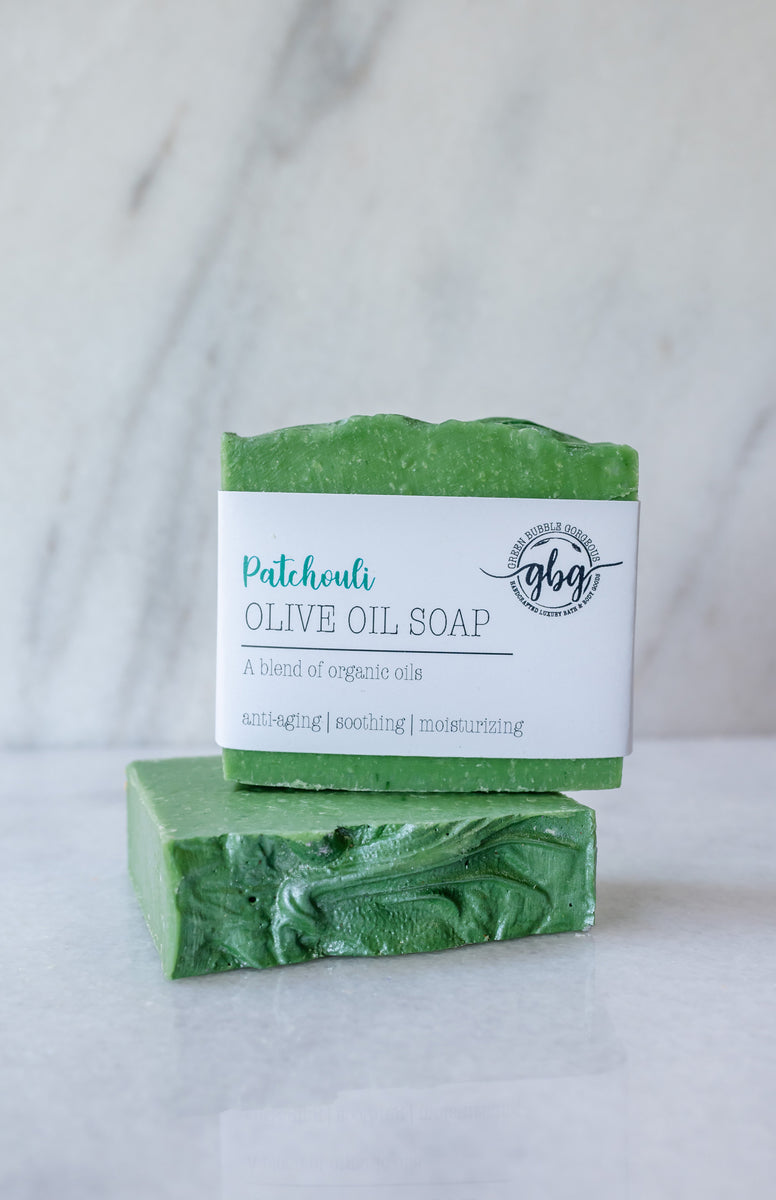The image features two bars of light green waxy soap identified as Patchouli Olive Oil Soap from Green Bubble Gorgeous (GBG), a luxury bath and body goods company. The soap bars, handcrafted from a blend of organic oils known for their anti-aging, soothing, and moisturizing properties, are stacked on a white marble surface with black flecks. One bar lies flat while the other stands upright on top, revealing a jagged edge that suggests they were once a single piece. The soaps are wrapped in a white paper label marked with the GBG logo, which includes "Green Bubble Gorgeous" in cursive and "Handcrafted luxury bath and body goods" in blocked letters encircling "GBG." The background, rendered blurry, also appears to be marble, creating an elegant and cohesive setting for the product.